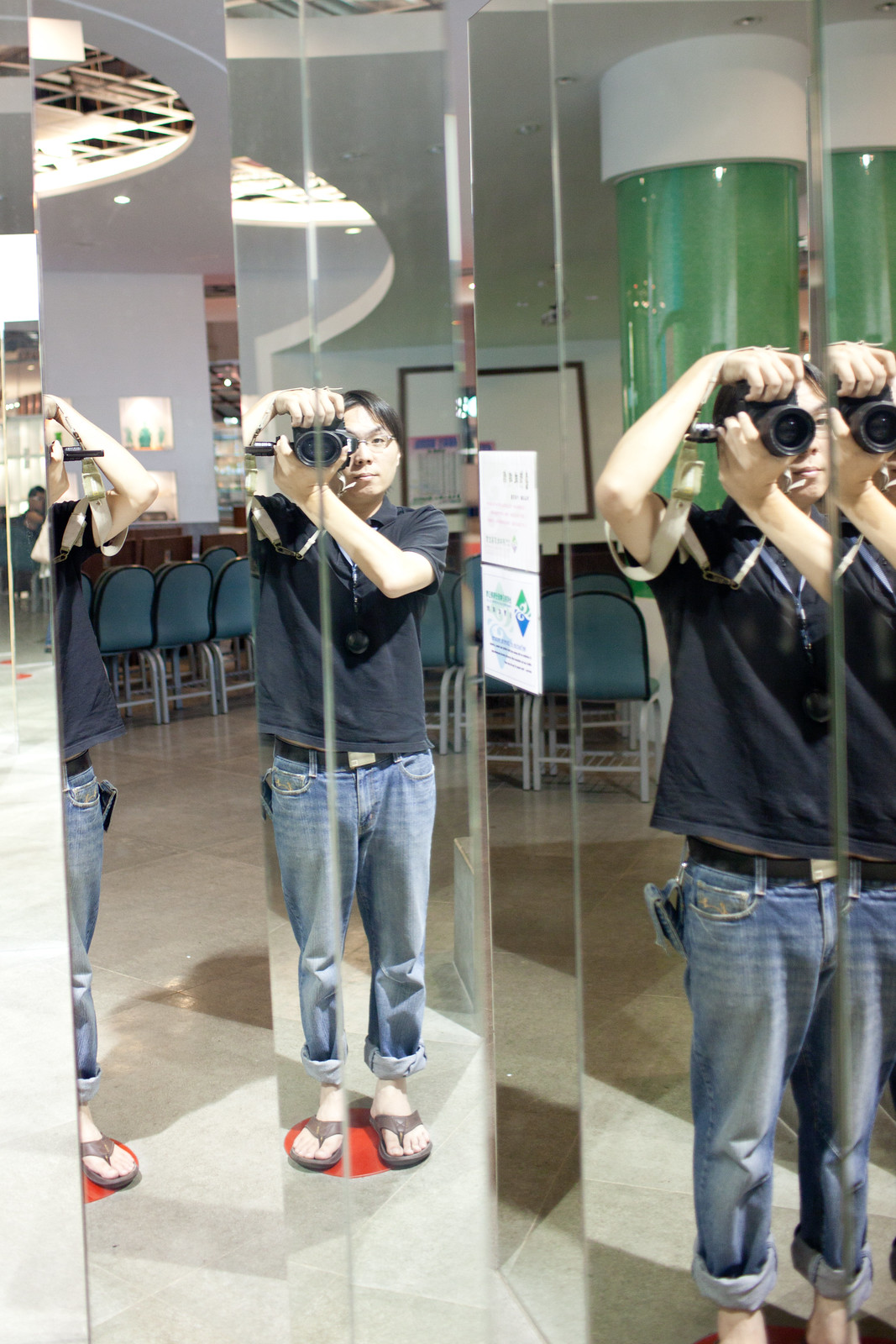In this color photograph taken inside a mall or a similarly public place, an Asian gentleman can be seen standing in front of a set of multiple, angled mirrors, capturing his reflection with a professional-looking, old-style camera held up to his right eye, our left. He is dressed in a navy blue polo shirt, cuffed blue jeans secured with a black belt, and brown leather flip-flops. His hair is dark brown, and he wears small glasses.

His posture, with arms slightly raised to steady the camera, creates an interesting reflection effect across the mirrors, resulting in three prominent reflections of him at varying angles. The backdrop features elements reminiscent of a hotel lobby or a convention center, including blue and black chairs, a large white tiled floor, a whiteboard, and a green column. The distorted reflections give the impression of a funhouse mirror setup, adding a playful touch to the overall composition. A red circle on the floor beneath him further anchors the scene.